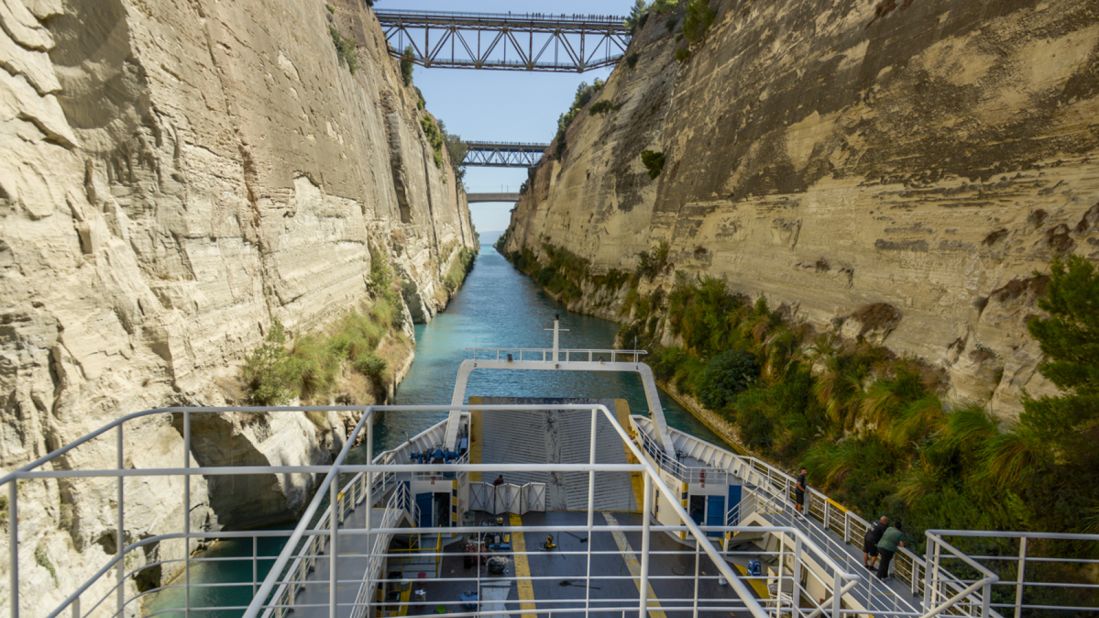The photograph depicts the viewpoint from the front deck of a ship navigating through a narrow canal, possibly the Suez Canal, captured during daytime. On either side of the canal, towering, rugged cliffs of pale yellow and brown stone rise steeply, with sparse vegetation on the left and slightly more greenery on the right. Along the cliffs, three distinct suspension bridges span from one side to the other, with the highest situated prominently in the foreground and the remaining two progressively farther in the background.

In the foreground, the ship's deck, composed predominantly of gray-painted metal, features several structural elements including pipes, railing, and tubing. Visible on the deck are two individuals: a couple standing together gazing at the right-hand cliff, and a lone figure a short distance away also observing the scenery. The teal blue water of the canal is flanked by the rocky cliffs, and in the far distance, there's an opening where the cliffs seem to part, revealing a hint of the sky above which is clear with a subtle haze near the horizon.